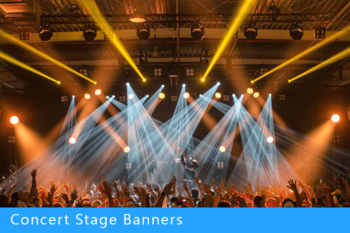This is a vibrant color photo of a concert scene. At the bottom, a blue banner with white text reads "Concert Stage Banners." From the ceiling, multiple stage lights project beams across the scene: six streams of yellow light stretch straight across, while blue lights illuminate different parts of the stage. On either side of the stage, an orange light points into the crowd, bathing the audience in a warm glow. The crowd itself is a sea of raised arms, though individual faces are indistinguishable. The stage is partially obscured, with only faint outlines and dark figures—likely the band members—visible through the dazzling lights. The atmosphere suggests a high-energy performance, with one performer on stage appearing to be passionately singing, arms raised high.